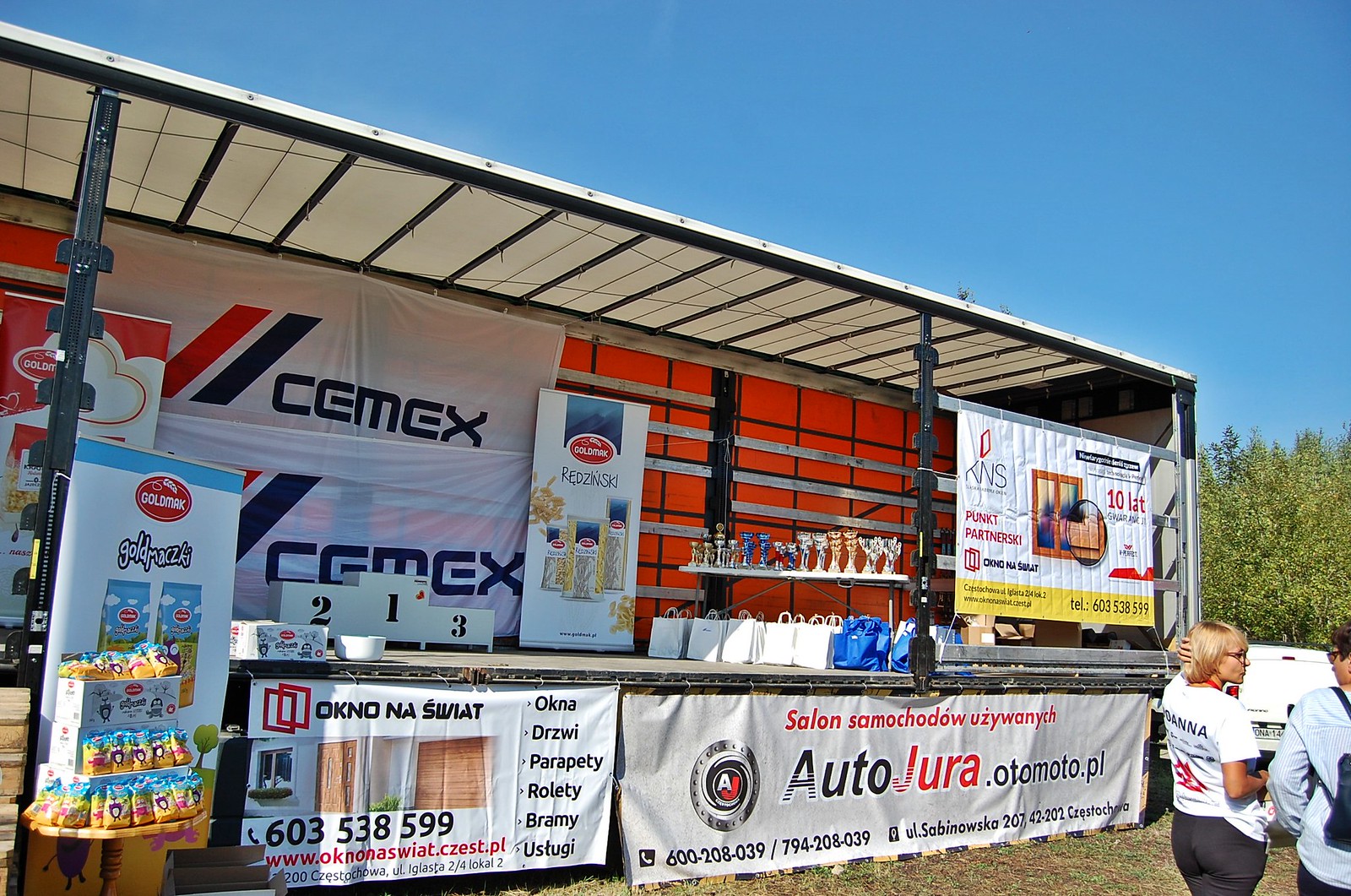The image depicts an outdoor festival or event on a clear, blue-sky day. The central focus is a large, elevated stage featuring a sturdy metal framework with lightweight top panels providing shade. The stage is positioned diagonally across the image, causing it to appear smaller as it extends to the right. Prominently displayed on the stage are three numbered platforms (1, 2, and 3), typically used for awarding first, second, and third place winners. In the middle of the stage, there's a white fold-out table laden with trophies and bags underneath. At the front of the stage, a series of banners hang, obscuring the space beneath. 

To the right, two people are standing on a grassy area in front of the stage, partially backed by a row of tall bushes. One person wears a white shirt with black text and a red logo, black pants, and has blonde hair. This individual has one hand on their head and is conversing with another person in a white long sleeve shirt. Additional features include a snack table on the left side of the stage with some items possibly being sold. The stage and surrounding area are adorned with various banners, including ones labeled "CEMEX" and "Goldmark Redzynski."